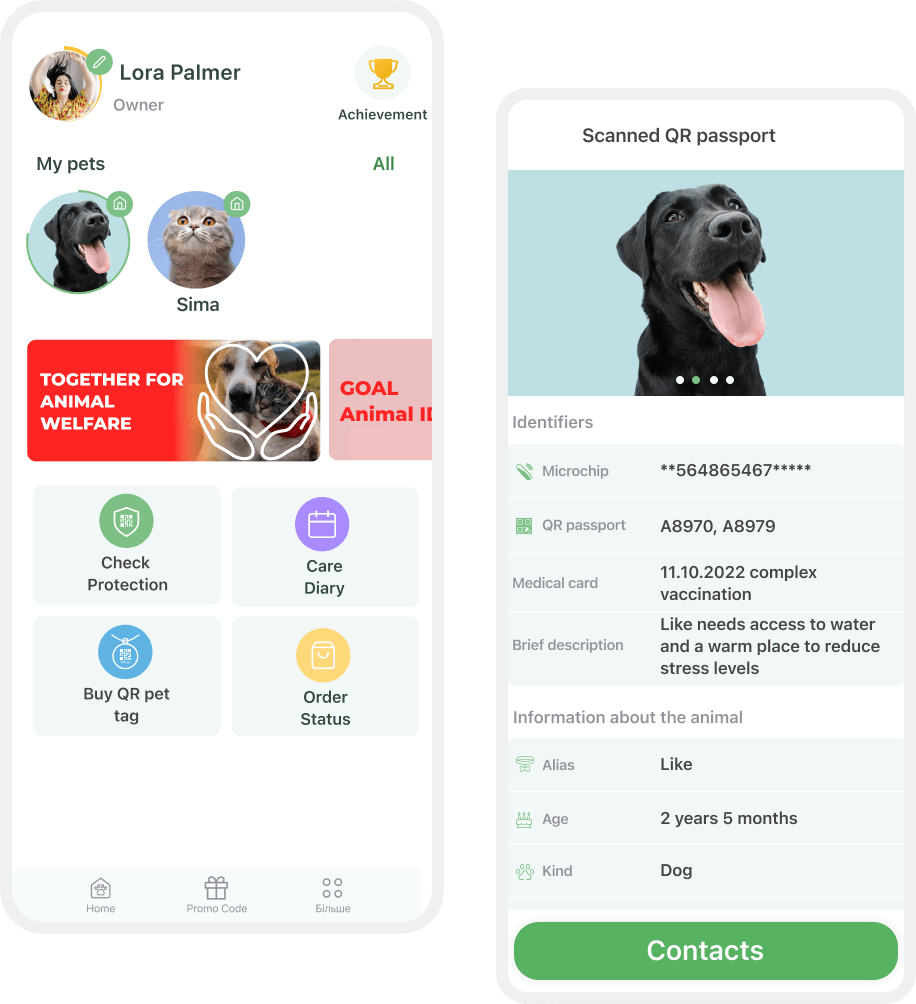### Detailed Descriptive Caption:

The promotional image showcases the various features of a pet-centric phone app designed for cat and dog owners. The layout consists of two distinct screenshots side by side.

**Left Screenshot:**
- The primary focus is on Laura Palmer, identified as an "Owner."
- Her profile includes two pets, a dog and a cat named Sima.
- A banner ad titled "Together for Animal Welfare" suggests an achievement or initiative related to animal care.
- Four functional buttons are prominently displayed:
  - **Check Protection**
  - **Care Diary**
  - **Buy QR Pet Tag**
  - **Order Status**
- The bottom navigation bar offers additional options:
  - **Home**
  - **Promo Code**
  - A button with Cyrillic text, likely related to the app's functionality but not translated into English.

**Right Screenshot:**
- This view displays the "Scanned QR Passport" of a dog, emphasizing the app’s capability to store crucial identification and medical information.
- Key features included:
  - **Identifiers** (Microchip number provided)
  - **QR Passport** (QR Passport number listed)
  - **Medical Card** with recent vaccination details dated 10-11-2022, mentioning "Complex Vaccination."
  - **Redescription:** Offers tips like the necessity for water and a warm place to mitigate stress levels.

- Additional animal details:
  - **Alias:** Like
  - **Age:** 2 years, 5 months
  - **Kind:** Dog
  - A **Contacts** button suggests quick access to contact information related to the pet's care.

Overall, the app appears to be a comprehensive tool for pet owners, consolidating pet identification, medical records, and welfare information into a single user-friendly interface.